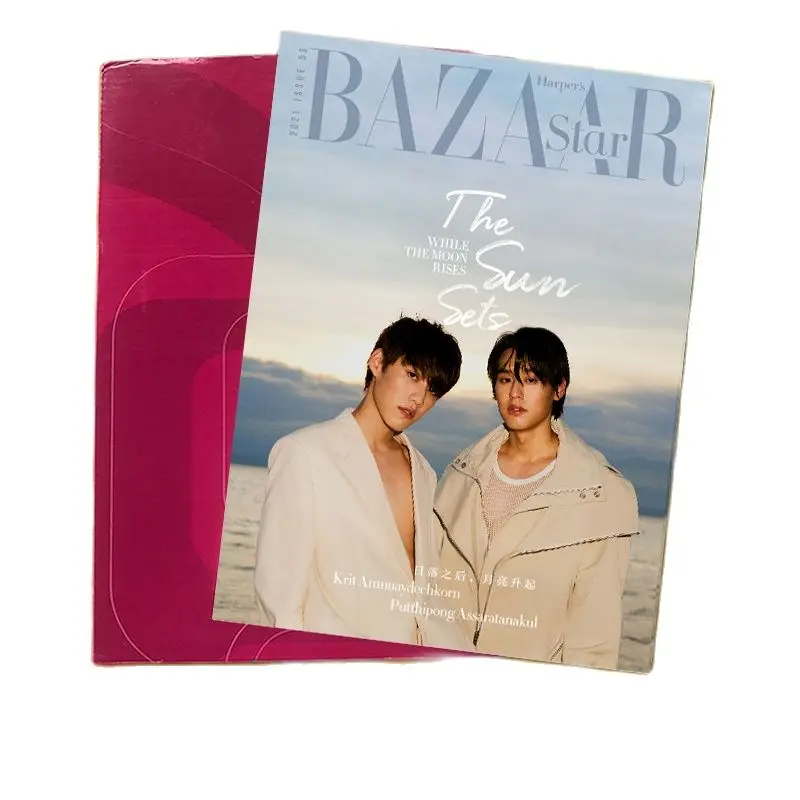The image is a cover of Harper's Bazaar magazine titled "Bizarre Star." At the top in gray text, it reads "2021 Issue 53," and beneath it, in white script, the caption says "the sun sets while the moon rises." The photograph features two Asian male models standing against a backdrop of a mountain range fading into a light blue-gray sky, with the sun setting behind clouds over a body of water. Both models have slightly long black hair falling to their ears and are looking directly at the camera. 

The model on the left is wearing a suit jacket with no shirt underneath, while the model on the right is dressed in a light-colored leather jacket paired with an off-white, wide-collared mesh shirt. They are dressed in cream hues and appear to be wearing lipstick. Below them, their names are displayed in Asian characters, with somewhat readable Latin alphabets indicating difficult-to-pronounce Thai names. The letters "Krit A-M-M-U-A-V-D-E-C-H-K-O-R-N-P-U-T-T-H-I-P-O-N-G-A-S-S-A-R-A-T-A-N-A-K-U-L" are partly visible at the bottom.

To the left of the cover, there is another rectangular shape, either magenta or maroon, featuring a pattern, slightly tilted and possibly just a piece of cardboard. The cover is set against a white background.